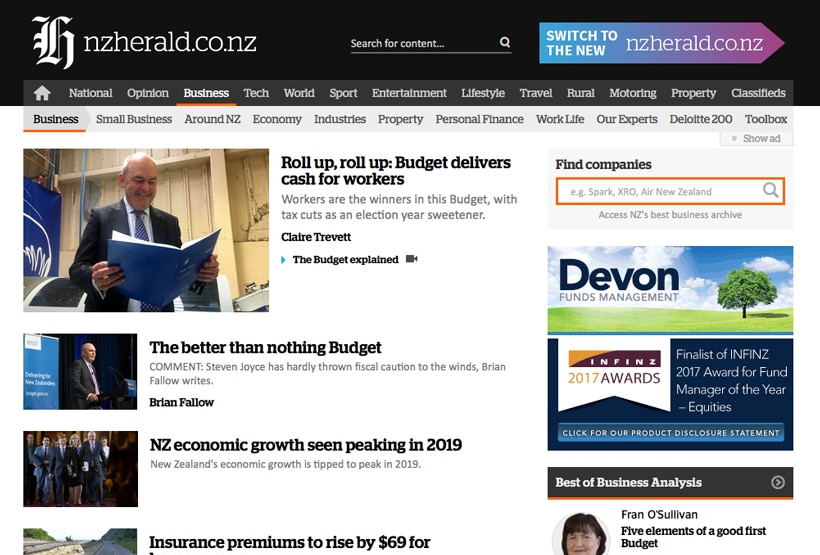This image captures a webpage from the New Zealand Herald's website, specifically the Business section. In the top left corner, the New Zealand Herald icon is prominently displayed along with the URL "nzherald.co.nz." Adjacent to this icon is a search bar labeled "Search for Content," featuring a small hourglass icon. To the right of the search bar, a notification box with a gradient from light blue to purple announces an upcoming switch to a new version of the website, "new.nzherald.co.nz."

Below this header, a horizontal grey tab bar lists various topics in white text from left to right: Home (with a house symbol), National, Opinion, Business (highlighted in white and underlined in orange), Tech, World, Sport, Entertainment, Lifestyle, Travel, Rural, Motoring, Property, and Classifieds. The Business section is currently selected, as indicated by the underlined tab.

Beneath the main topics tab, a subtopics bar in light grey with black text lists additional categories: Business (again underlined in orange), Small Business, Around NZ, Economy, Industries, Property, Personal Finance, Work Life, Our Experts, Deloitte 200, and Toolbox.

The main part of the page features several articles with accompanying images. The largest image on the top left depicts a man in a black coat, grey tie, and white shirt looking down at a blue folder while smiling. His balding head with hair on the sides is clearly visible. Adjacent to this image, the headline reads: "Roll Up, Roll Up Budget Delivers Cash for Workers" with the subheading, "Workers are the winners in this budget with tax cuts as an election year sweetener by Claire Trevett." Below this subheading, a video icon accompanies the text "The Budget Explained."

The subsequent articles include:
- "The Better Than Nothing Budget," a commentary with a single comment, written by Brian Fallow.
- "NZ Economic Growth Seen Peaking in 2019," which discusses the anticipated peak in New Zealand's economic growth that year.
- The final partially visible article titled "Insurance Premiums to Rise by $69.04," with the rest of the title cut off.

On the right-hand side of the page, there is a "Find Companies" search box highlighted with an orange outline. Below this search box, three advertisements are displayed: 
1. Devon Funds Management.
2. Infini's 2017 Awards.
3. Best of Business Analysis featuring Fran O'Sullivan's "Five Elements of a Good First Budget."

Overall, this image provides a detailed snapshot of the Business section of the New Zealand Herald's online platform.